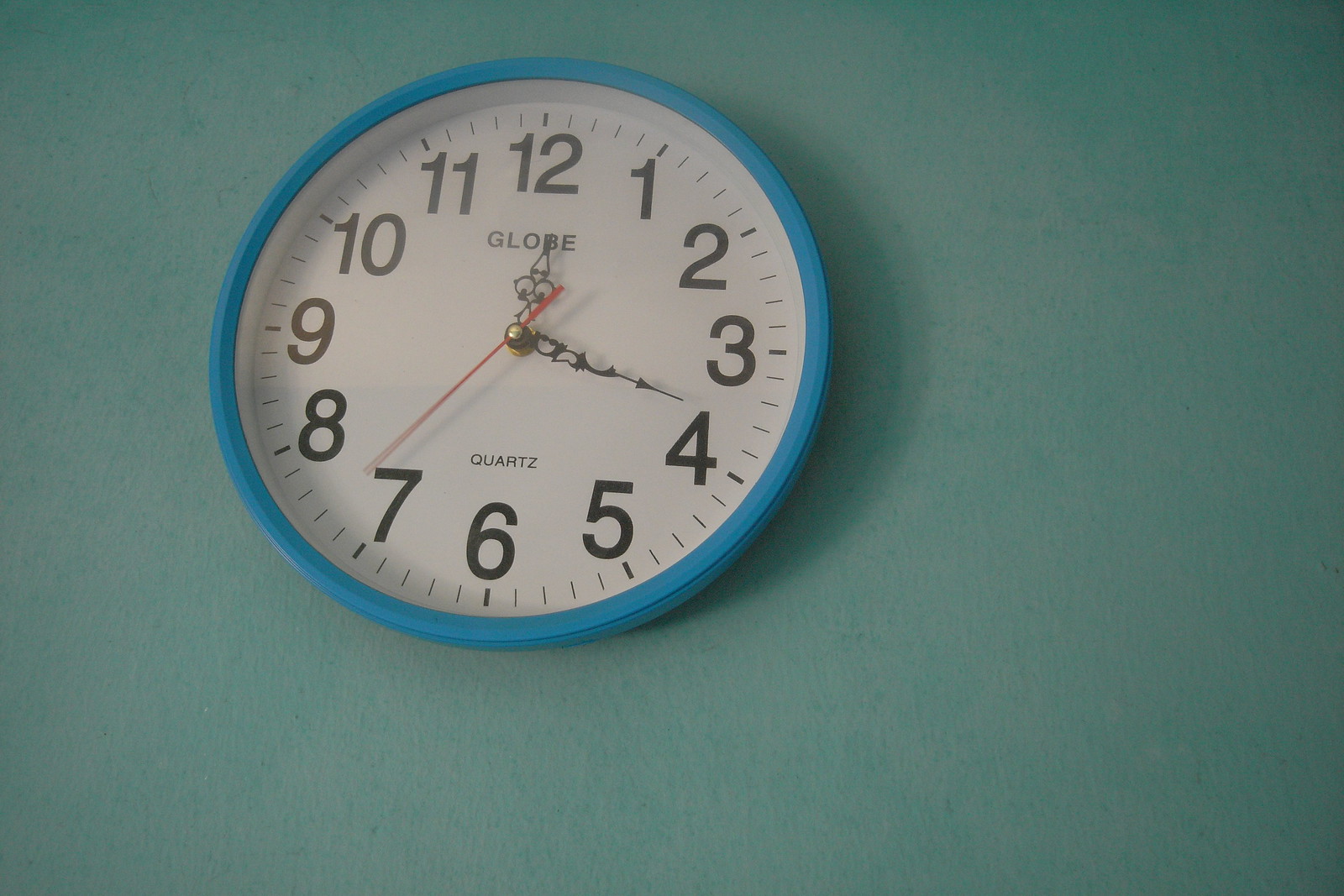This photograph features a classic circular analog quartz wall clock with a white face and standard black numerals ranging from 1 to 12 in a common font. The brand "Globe" is prominently displayed on the clock face. The second hand is distinctively red, while both the hour and minute hands are ornate black. Encircling the clock face is a light blue plastic bezel. The clock is mounted on a greenish-gray wall, giving the impression of a familiar classroom setting, likely positioned above an instructional board. The straightforward design and the functional elements make it a quintessential example of a typical wall clock found in educational environments.